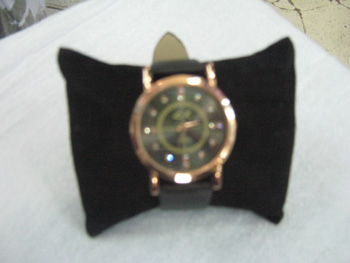The somewhat blurry image captures a black watch with a gold frame, elegantly strapped to a small black pillow. The watch's face is black, adorned with what appears to be gold hands and possibly gold numbers or Roman numerals, though the blur makes it hard to distinguish. This plush black pillow sits close to the edge of a white surface, likely a table, with the surface of a concrete floor visible in the background. The concrete floor appears cracked, with some of the fissures visible in the upper right-hand corner of the image. The white table and cracked concrete floor hint at an environment that juxtaposes the watch's refined elegance with a more rugged and worn setting.